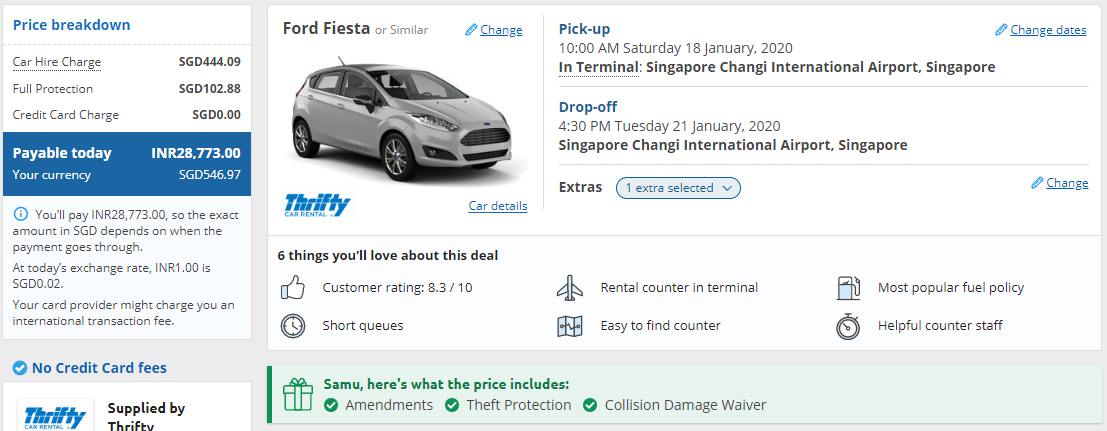The image depicts a web page from the Thrifty website, showcasing a vehicle, namely a gray Ford Fiesta. The Thrifty logo, featuring a blue design, is prominently visible twice: once in the bottom left corner and again in the center left of the image. At the top left, the vehicle model "Ford Fiesta" is displayed.

The context suggests that this vehicle is available either for rental or purchase, with more indications leaning towards a rental service. In the top right, there is a section labeled "Pickup" with details underneath: the scheduled pickup time is 10:00 a.m. on Saturday, January 18th, 2020, located at Singapore Changi International Airport, Singapore. Below this, another section labeled "Drop-off" indicates the vehicle is to be returned at 4:30 p.m. on Tuesday, January 21st, 2020, at the same airport.

The detailed information implies this is likely a rental service being described on the Thrifty website, specifically for the Ford Fiesta.